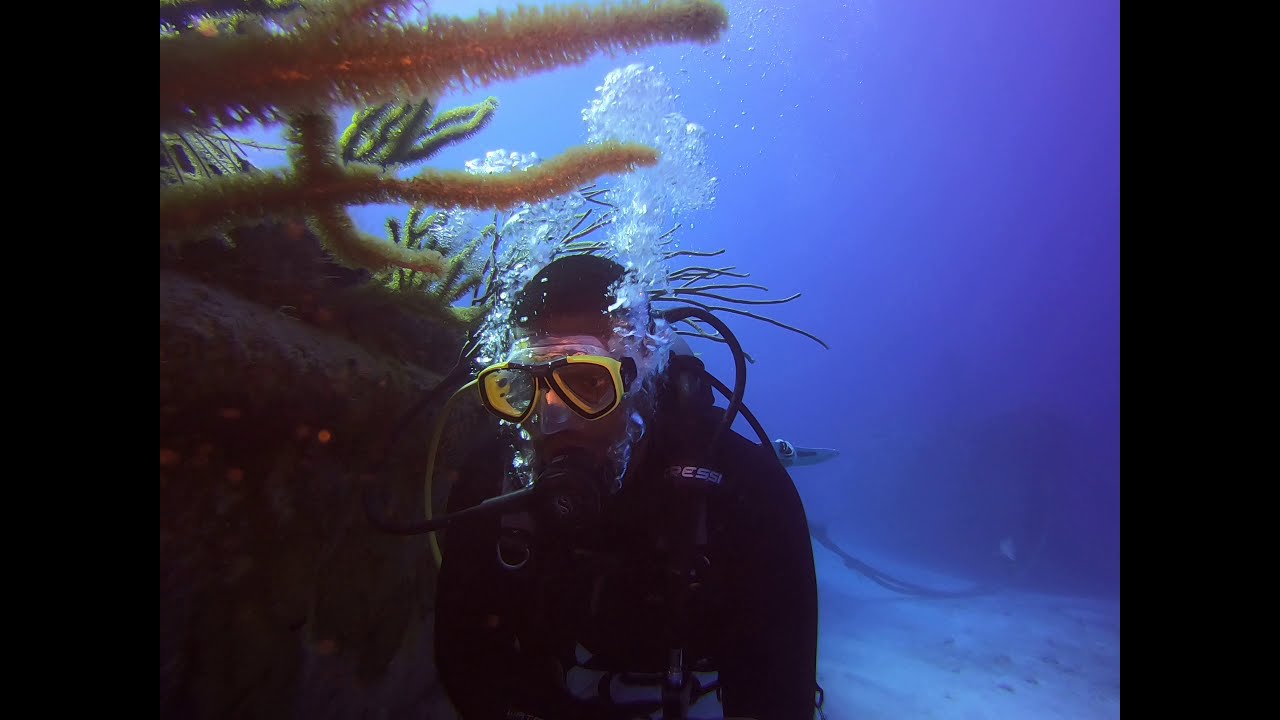A dark-skinned man is scuba diving in the depths of a vibrant blue ocean, positioned centrally in the image. He is equipped with a full set of scuba gear, including large yellow goggles and a black breathing apparatus in his mouth, all complementing his black outfit. Bubbles rise from his mouthpiece, journeying upwards through the water. His body is oriented forward, with his gaze directed slightly downward to the side. To the left side of the image, a series of green and yellow underwater plants grow behind a small brown rock formation. The ocean behind him fades into a bright blue expanse, creating a serene yet lively scene.